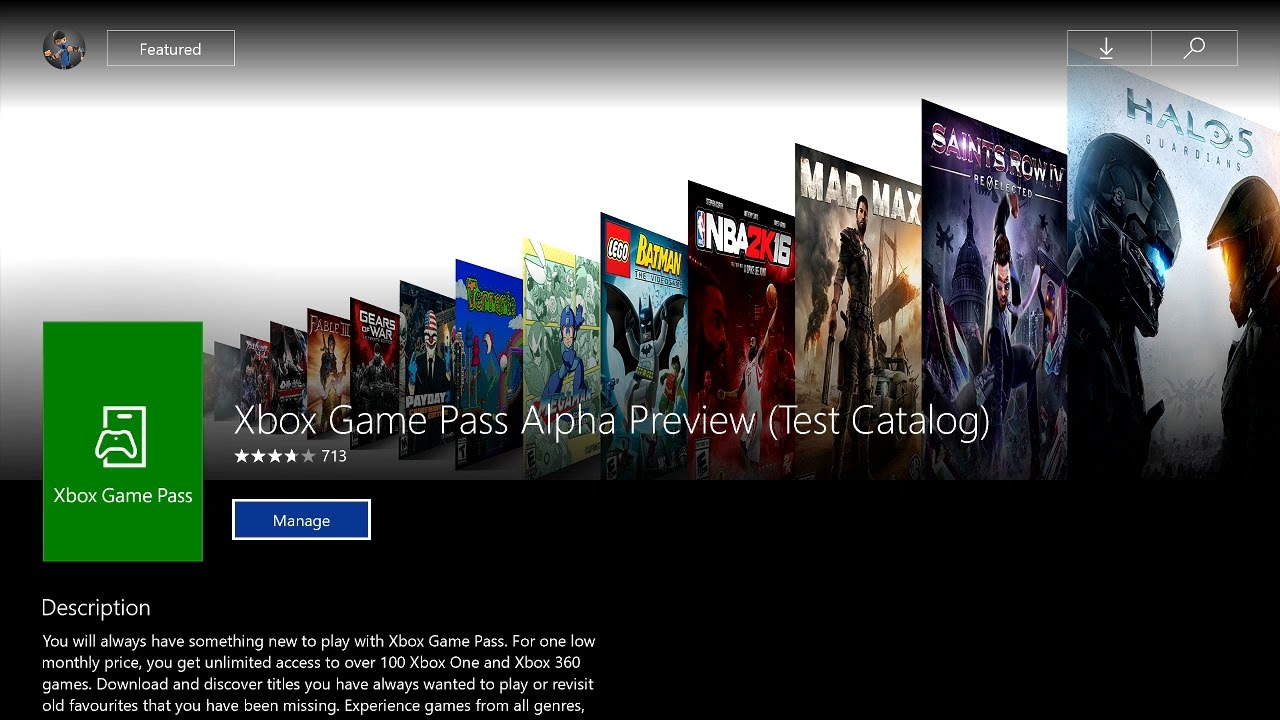The screenshot appears to be from the Microsoft Store interface. At the top, there's a circular avatar, possibly representing the user's profile. Adjacent to the avatar, you see a "Featured" button, a download button denoted by a downward-facing arrow, and a search icon represented by a magnifying glass.

Dominating the header is a collage of various game covers, overlapping one another. A green banner prominently displays "Xbox Game Pass" along with a simplified Xbox console icon. The text reads "Xbox Game Pass Alpha Preview (Test Catalog)", suggesting an early access feature for testing purposes. The service holds a rating of approximately four stars, accumulated from 713 reviews.

A noticeable blue button labeled "Manage" in white text stands out beneath the header. This is followed by descriptive text, starting with a heading labeled "Description". The readable portion of the description states: "You always have something new to play with the Xbox Game Pass for one low monthly price. You'll get unlimited access to over 100 Xbox One and Xbox 360 games. Download and discover titles you have always wanted to play or revisit old favorites that you have been missing. Experience games from all genres..." The text is truncated at this point.